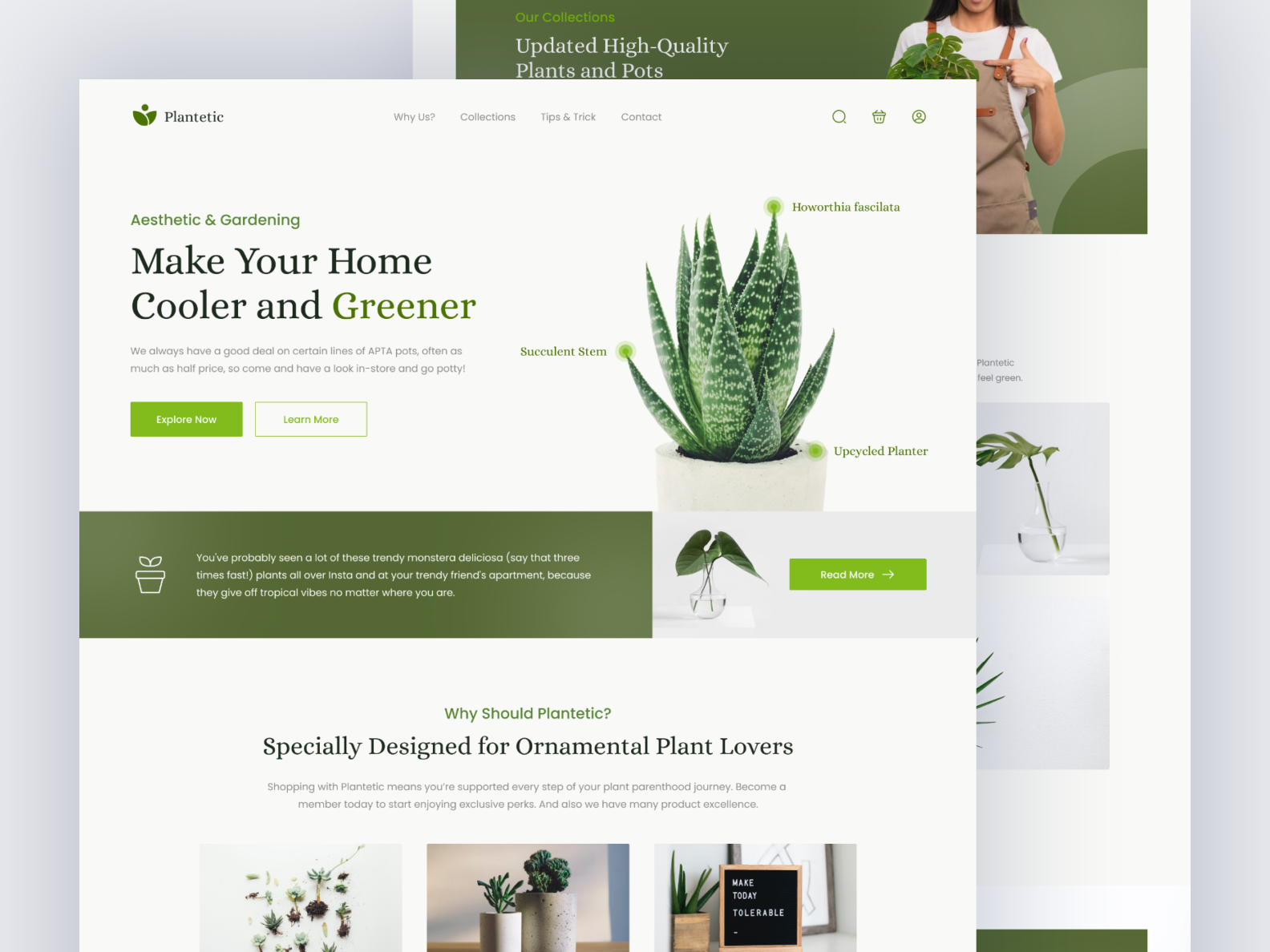The image depicts a webpage for "Plantetic" with a light gray background featuring two overlapping screens. The foremost screen prominently displays the Plantetic logo, consisting of the company name in the top left corner alongside a small plant icon. Central elements of the screen include navigational links labeled "YS," "Collections," "Tips and Tricks," and "Contact." To the right, there are icons for search, trash, and login functionalities.

Below these elements is an image of a succulent annotated with circular markers identifying its parts: "Succulent Stem," "Haworthia Fasciata," and "Upcycled Planter." Adjacent to this image, text reads, "Make your home cooler and greener," with buttons labeled "Explore now" and "Learn more." Another caption on the left highlights Plantetic's appeal to ornamental plant enthusiasts with the words, "Specially designed for ornamental plant lovers."

The background screen, partially obscured by the foreground elements, features a top section titled "Our Collections, Updated High Quality Plants and Pots." This screen has a green background and depicts a woman standing on the right side wearing overalls. She holds a Monstera plant and gestures towards it, suggesting the variety and quality of the plants offered by Plantetic.